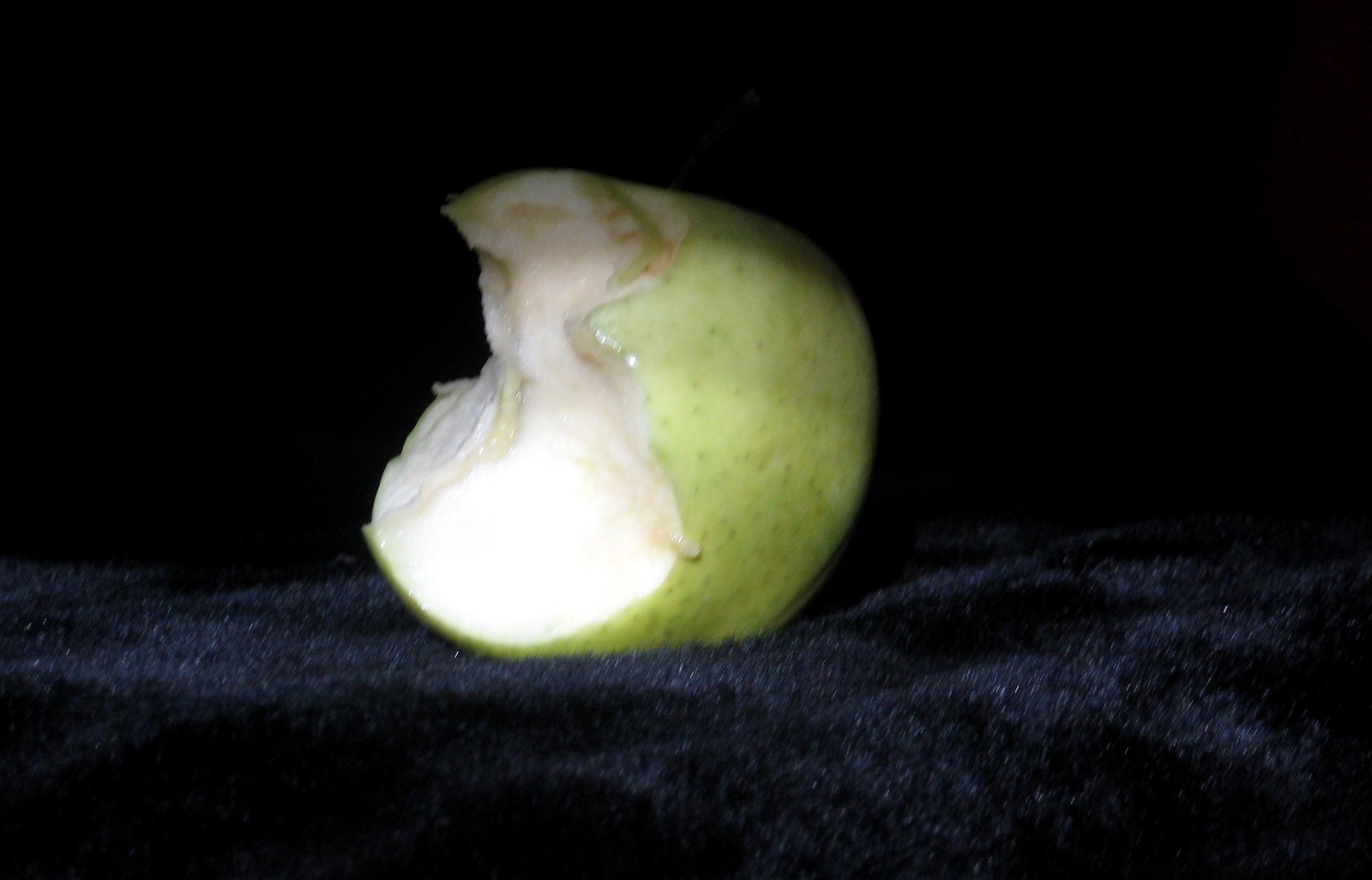A partially consumed green apple, characterized by its pale green skin with darker green specks, sits against a backdrop of luxuriously draped black velvet fabric. Although the surroundings are dimly lit, a soft illumination from the top left subtly highlights the apple, punctuating its position within the otherwise shadowy scene. The apple reveals large, jagged bite marks, with about two-thirds of its form remaining. The exposed flesh is predominantly white, though the area around the topmost bite exhibits slight browning. Through the blurred core, denser fibrous material is visible, hinting at the apple's inner structure. Glistening moisture adorns the surface of the apple, enhancing its textured appearance amidst the deeply shadowed, almost ethereal setting—perhaps a conceptual start to a still life study.